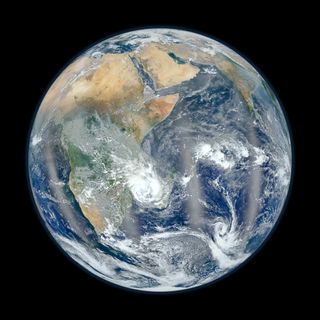This color photograph captures a stunning view of Earth from space, revealing the vastness of our planet against a black backdrop. The entire photograph is framed in a square orientation, emphasizing the spherical nature of Earth against the surrounding void of space. Prominently featured in the image is the continent of Africa, depicted with sub-Saharan Africa in vibrant green hues and the remaining land in brownish tints. 

To the northeast of Africa, the Arabian Peninsula extends into the Middle East, showcasing a comprehensive view that includes regions all the way to Pakistan and the entire Indian subcontinent. The bottom part of the globe provides a glimpse of Antarctica, characterized by swirling white cloud formations. The Earth's oceans are a vivid blue, contrasting with the various land masses that exhibit shades of brown and green.

White cloud formations are visible throughout the atmosphere, creating marble-like swirls that provide a dynamic texture across the globe. The interplay between the blue oceans, brown and green landmasses, and the white clouds gives Earth a mesmerizing, almost marble-print appearance. The photograph effectively conveys the sheer scale and beauty of the planet, with its diverse geographical features and the serene blackness of space surrounding it.